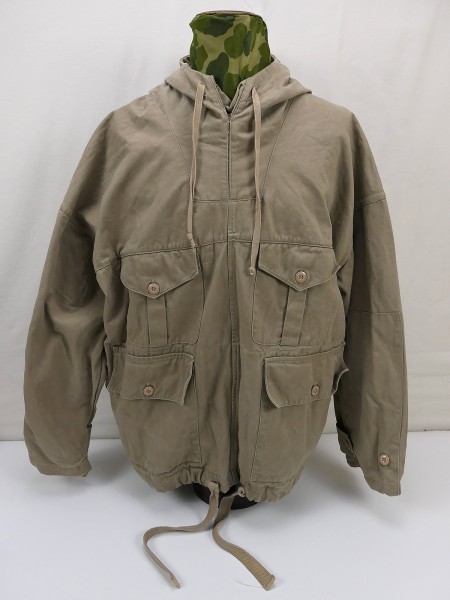The photograph features a beige, light brown jacket displayed on a headless, half-mannequin torso with a camouflage-like material draped over it. The setting has a white floor and a white wall background, creating a neutral environment that highlights the jacket. The jacket, which is zipped up to the top, boasts a hood with drawstrings and distinctive features such as four front pockets arranged in two rows beneath the breast area. The upper pockets have central pleats, while the larger lower pockets include flaps and side openings. Additional details include drawstrings at the bottom and around the neck, both untied, and buttons at the wrists of the drop-shoulder sleeves.